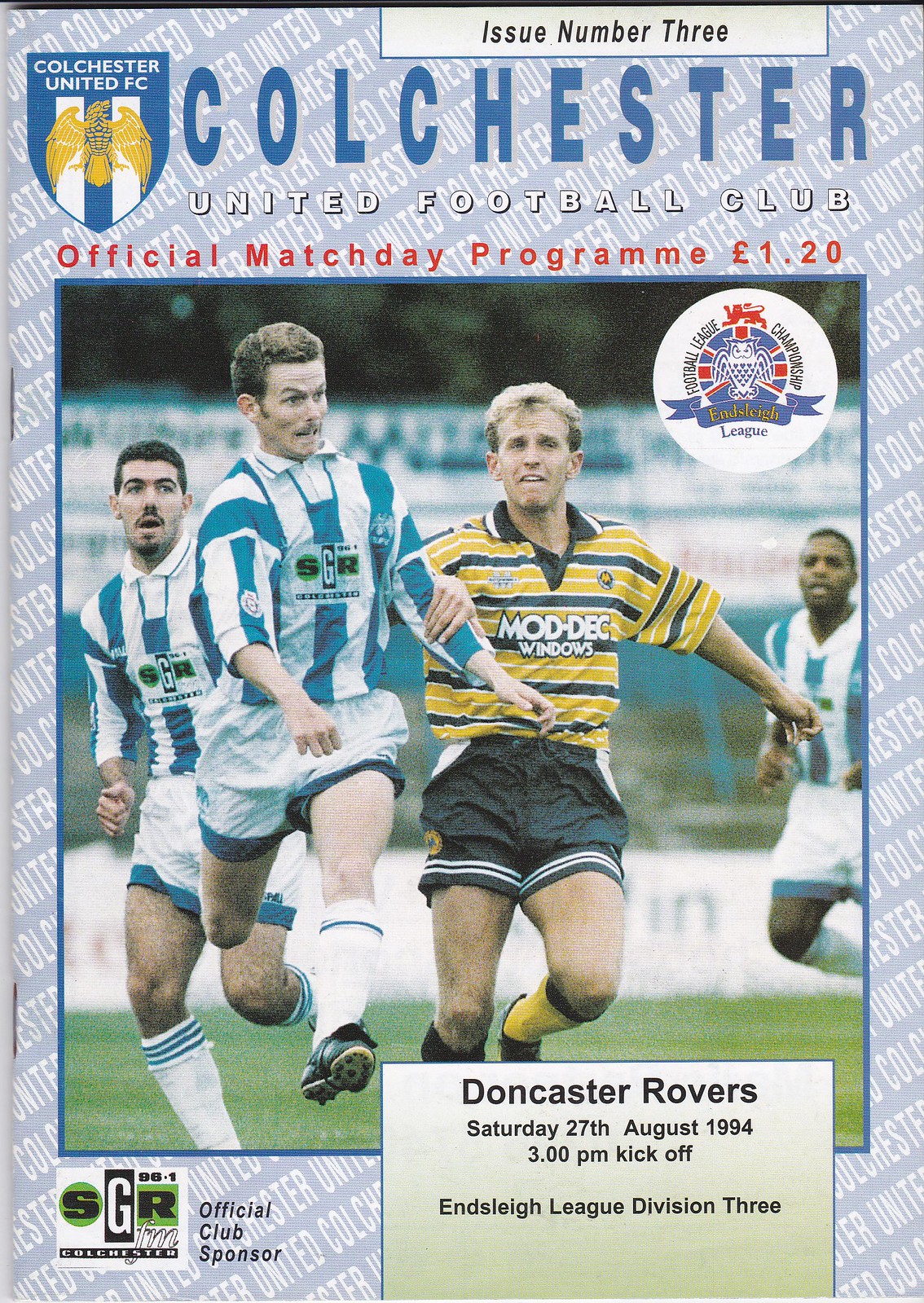On the cover of this vintage Colchester United Football Club official match day program, identified as Issue Number Three, dated Saturday, August 27, 1994, and priced at £1.20, a dynamic photograph prominently features four soccer players in action. The players, dressed in Colchester's traditional blue and white vertical-striped jerseys with white shorts accented by blue trims, are captured mid-game against an opposing team in yellow and horizontal white and blue stripes. Above the image, the program's title is segmented into three color-coded sections: "Colchester" in bold blue text, "United Football Club" in striking white letters, and "Official Match Day Program" in vivid red text. An eagle emblazoned on a flag-like shield, the club's emblem, is positioned top left of the cover. Towards the bottom right, essential match details such as "Doncaster Rovers," "Saturday 27th August 1994," "3 p.m. kickoff," and "Ensley League Division III" are clearly stated in black text. To the left, the program also acknowledges the official club sponsor, SGR.